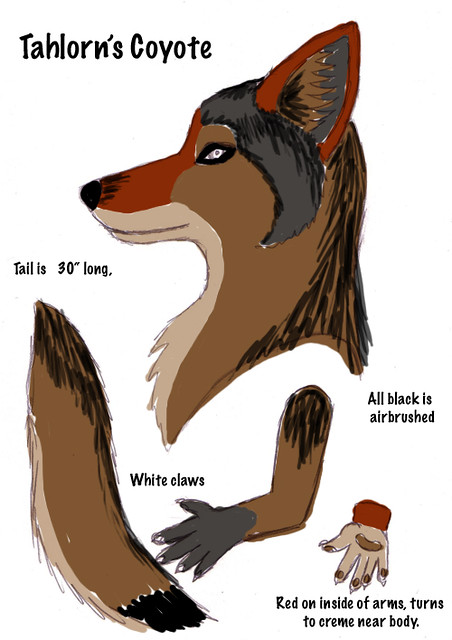This is a detailed, somewhat amateur-styled exhibit, possibly a school project, featuring a segmented depiction of a coyote. The heading at the top left reads "Taylor's Coyote" in informal, capitalized lettering. The central focus is the coyote's head, directed to the viewer's left, showcasing a mix of black, brown, and tan fur, and a black nose with a red tint on the snout. The coyote has a wide-open mouth with no visible teeth and a side profile showing one ear, which is red-lined with black and brown in its inner area. Strikingly, two black crescent swooshes near the eye give the appearance of eyeliner. 

The lower left corner displays the coyote's tail, labeled "Tail is 30 inches long." The tail features a color gradation from black at the top, through brown in the middle, to tan at the bottom, with a black tip. Adjacent to the tail is a disembodied, bent arm with a white-clawed paw; the arm is black at the top, brown in the middle, and gray near the paw. Above the paw, text reads "White claws."

On the lower right of the head, there’s printed text stating "All black is airbrushed." Furthermore, there is an illustration of the underside of the coyote's paw, tan with a mahogany stripe, and a centered red-print label that reads, "Red on inside of arms turns to cream near body."

Overall, the image features an array of colors including red, black, browns, light browns, grays, and whites, contributing to the illustrated segments of the coyote and detailed descriptive annotations.